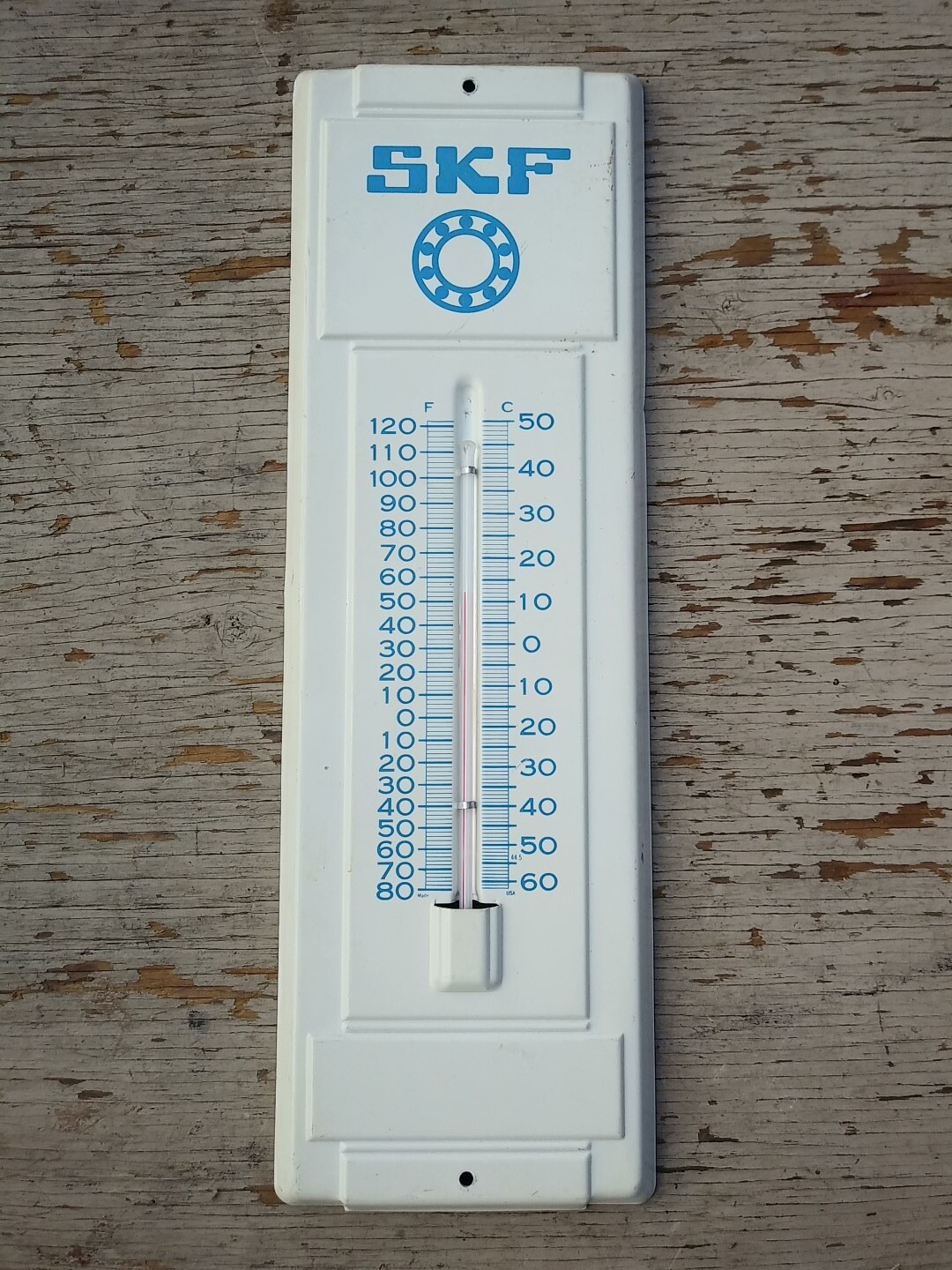This image shows a close-up of a white rectangular thermometer placed on a wooden surface, highlighting its detailed features. The wooden surface exhibits two shades of brown: the predominant hue is a medium brown interspersed with lighter brown stripes, and there are also darker brown areas where the stripes have been scratched off. Dominating the center of the image is a large white vertical rectangle, with a smaller horizontal rectangle positioned at the bottom.

At the top, "SKF" is inscribed in blue within another rectangle, accompanied by a circular logo directly underneath it. This logo features a series of dots around its perimeter and a smaller circle within. Flanking a small, thin glass tube filled with mercury, which measures the temperature, are vertical lines. The left side of the thermometer displays measurements in Fahrenheit (F), while the right side shows corresponding readings in Celsius (C). Each side has vertical numeric markings indicating temperature values respective to each scale.